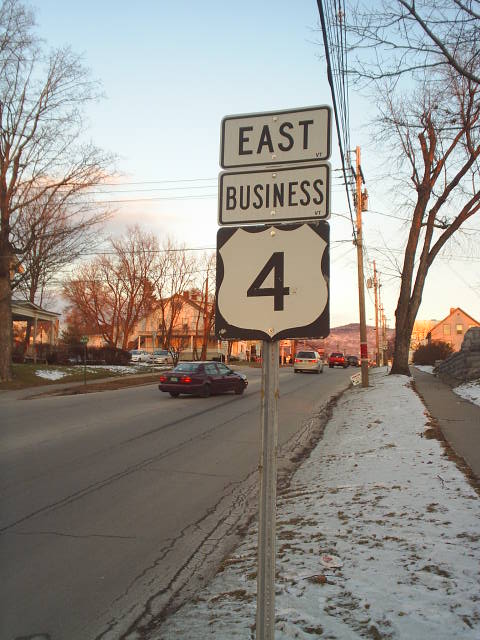The photograph captures a suburban street intersection with a prominent street sign in the foreground. This metal sign is composed of three distinct sections: the top section says "EAST" in black font on a white rectangular background, the middle section reads "Business" in black font on a similar white background, and the bottom section features a black number "4" on a white shield-shaped sign with a black outline, likely indicating U.S. Highway 4's business route. The sign is planted in a median of grass that's dusted with snow, separating it from the road and a nearby sidewalk.

Beyond the sign, several cars are visible, some appearing to turn left or head away from the viewer's perspective, their lights glowing dimly. The road is flanked by patches of snow-covered grass and dotted with bare trees, suggesting a wintry setting. In the background, a mix of houses and possible businesses line the street. One house is characterized by a large wraparound porch, while another structure appears more modern, potentially an apartment complex made of brown wood. The sky is clear, and sunlight brightens the area slightly further down the road. This serene, shaded suburban scene is framed by rows of leafless deciduous trees.